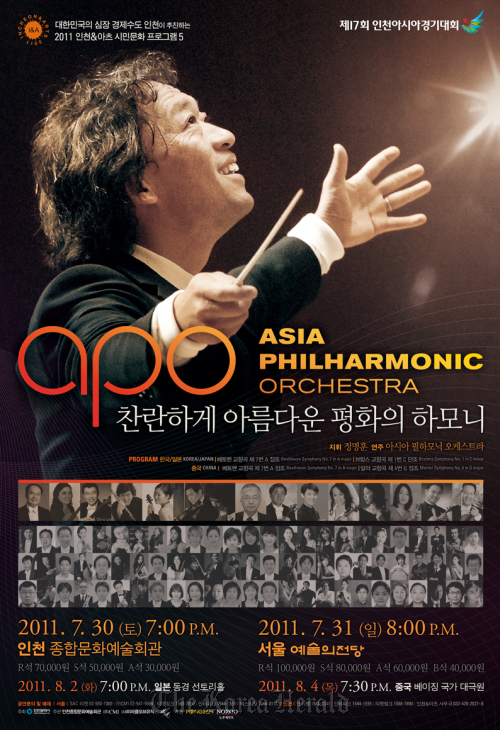The advertisement for the Asia Philharmonic Orchestra features a striking side-profile photograph of an Asian conductor, exuberantly poised in mid-performance. Dressed in a black suit with a white dress shirt, he holds a conductor's baton in his right hand, while his left hand splayed out energetically. His face, framed by black curly hair and a broad smile, tilts upward towards a bright light in the upper right-hand corner, suggesting a dramatic moment of musical triumph. The only English text on the poster reads "Asia Philharmonic Orchestra" in vibrant yellow and orange lettering, accompanied by the acronym "APO". Surrounding this are dense columns of Asian characters, presumed to be Korean. Beneath the conductor’s image, starting from shoulder level, are four rows of black and white photographs, each row containing about twelve individual images of orchestra members. At the bottom, the poster details performance dates and times in a mix of orange text and Korean script, advertising concerts on July 30, 2011, at 7 p.m. and July 31, 2011, at 8 p.m. The entire advertisement is set against a deep black background, enhancing the dramatic lighting and the conductor's expressive pose.